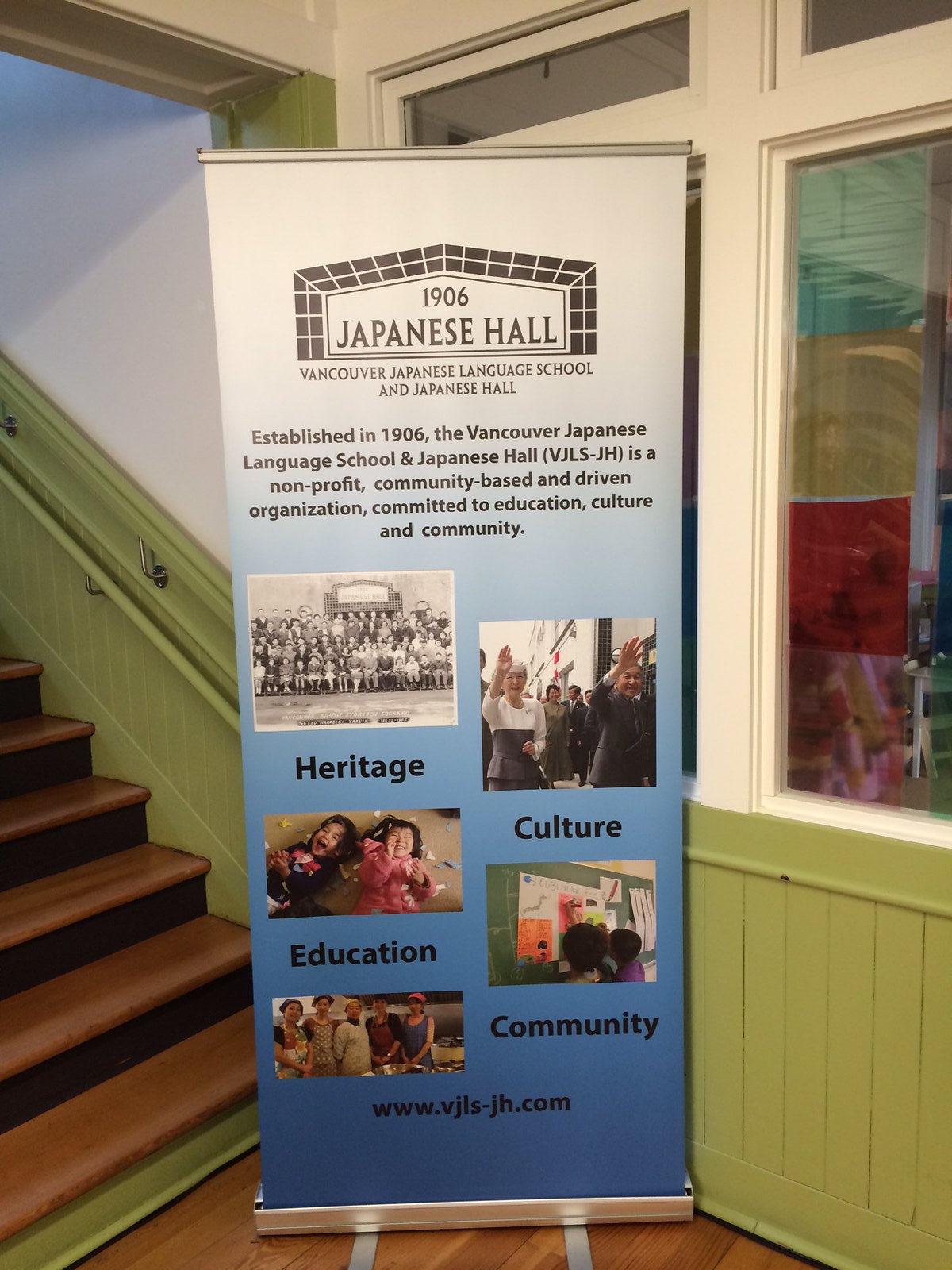This tall, rectangular indoor photograph showcases a prominently placed sign standing on a silver stand at the edge of a set of stairs. These stairs, positioned to the left and identified by their brown wooden steps and light green railings and sides, lead up through the scene. The green portion extends to the bottom right corner of the image, complementing the wooden floor that underscores the setting's natural hues.

The sign itself features a gradient from white at the top to blue at the bottom. Dominating the top portion is a black checkered symbol resembling a stage, encircled by the words "Japanese Hall" in bold black letters. Just below, in all capital letters, it reads "Vancouver Japanese Language School and Japanese Hall," immediately followed by a paragraph explaining the institution's foundations. The text describes the establishment of the Vancouver Japanese Language School and Japanese Hall (VJLS-JH) in 1906, detailing it as a non-profit, community-driven organization dedicated to education, culture, and community.

In the lower section of the sign, five images provide visual context. These include a black and white photograph labeled "Heritage," depicting a group; a photo of a man and a woman labeled "Culture"; an image of two small children marked "Education"; another picture of schoolchildren labeled "Community"; and, at the very bottom, a picture of a group of Asian women in a kitchen with the accompanying website "www.vjls-jh.com." The composition and captions collectively underscore the community's rich heritage and ongoing commitment to cultural education.